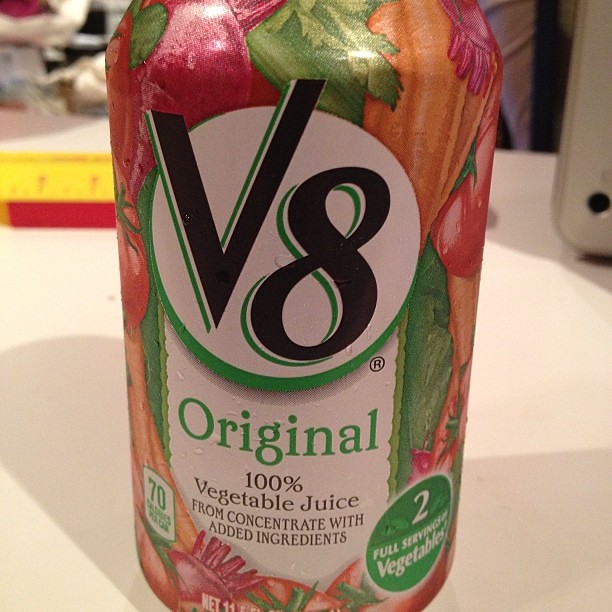The image captures a can of V8 juice prominently displayed on a white table. The front of the can features a large circular logo with 'V8' written in bold, followed by the word 'Original'. Beneath this, it states '100% Vegetable Juice from Concentrate with Added Ingredients'. To the left, the can indicates '70 Calories per Can', and to the right, a green circle highlights '2 Full Servings of Vegetables'. The can’s design is adorned with a vibrant mosaic of various vegetables, creating a visually appealing and nutritious impression. In the blurred background, the setting appears to be a bustling environment, potentially a classroom, filled with indistinct figures and activities, adding to the context without distracting from the focal point—the can of V8 juice.